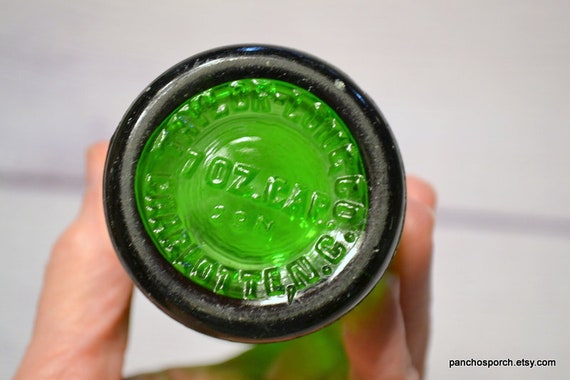This image captures a close-up view of a glass bottle being held by a person with visible three fingers and a thumb. The bottle has a distinctive design, with a jet black outer rim and a central section in a vibrant lime green color. The bottle's bottom surface features embossed text that partially reads "7 ounce cap," though other characters around it are hard to discern due to glare. The image also prominently displays the website "ponchosporch.etsy.com" at the bottom right corner. The background is predominantly white with a subtle gray line, and the focus is maintained sharply on the bottle, showcasing its details while blurring out the rest. The quality of the image is notably high, emphasizing the bottle's features and the clarity of the surrounding text.